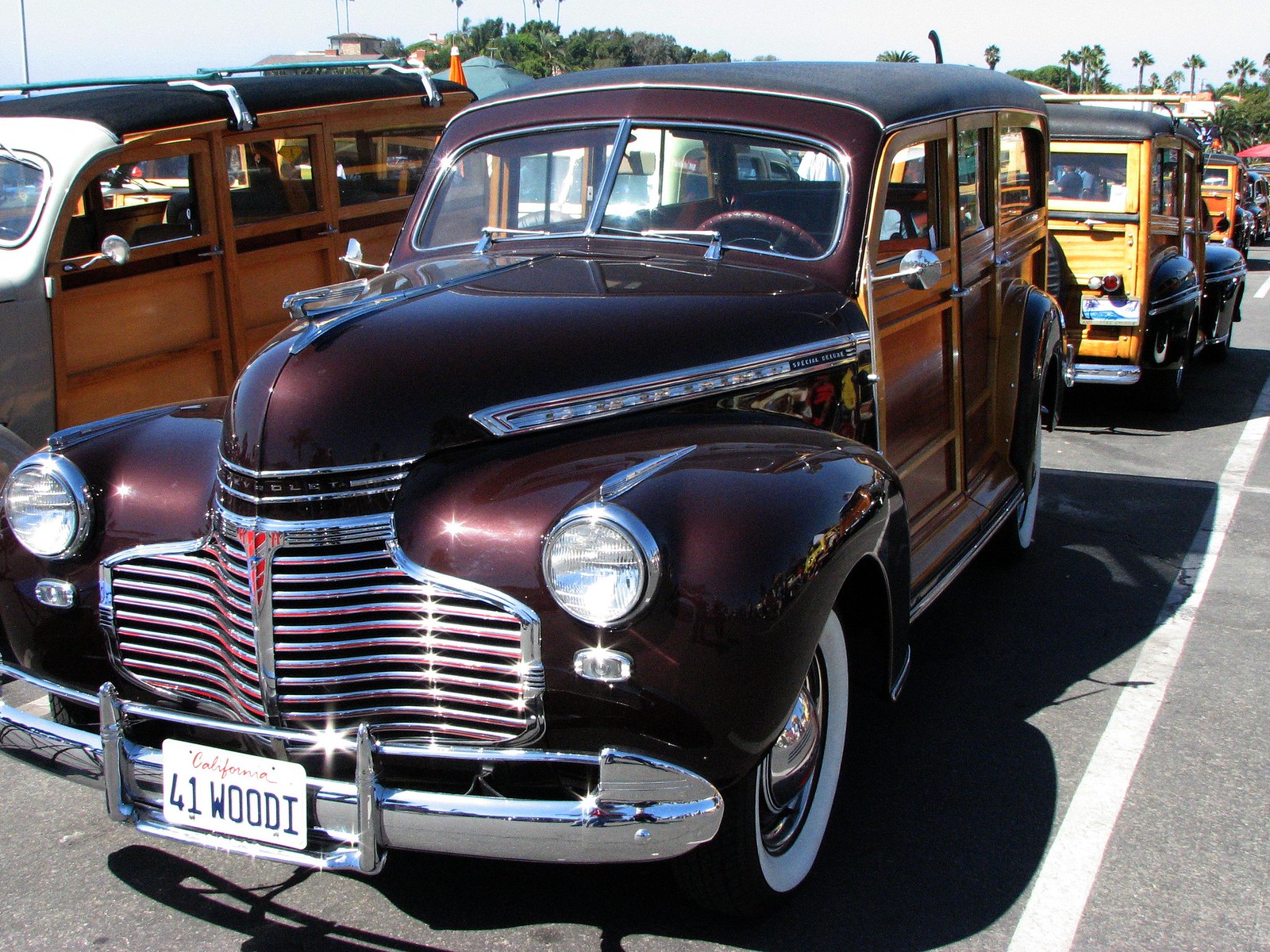In this color photograph taken on a sunny day, we see a large parking lot filled with beautifully restored vintage cars, suggesting it might be a classic car show. Dominating the foreground is a deep burgundy, 1941 Woody with a California license plate reading "41 W-O-O-D-I". It features wooden doors and side panels, along with chrome highlights, aligning with the classic Woody style. The vehicle is positioned almost straight-on to the photographer, giving a clear view of its long hood and intricate details. 

Around the burgundy Woody, there are several other classic cars, partially obstructed yet distinct in their vintage design. To the left, another car showcases similar wooden doors and side panels, while a yellow and black vehicle is visible behind the main subject. The well-maintained condition of these cars further emphasizes the possibility of a car-related event. Palm trees and a blue sky provide a quintessential California backdrop, enhancing the nostalgic atmosphere of the scene.